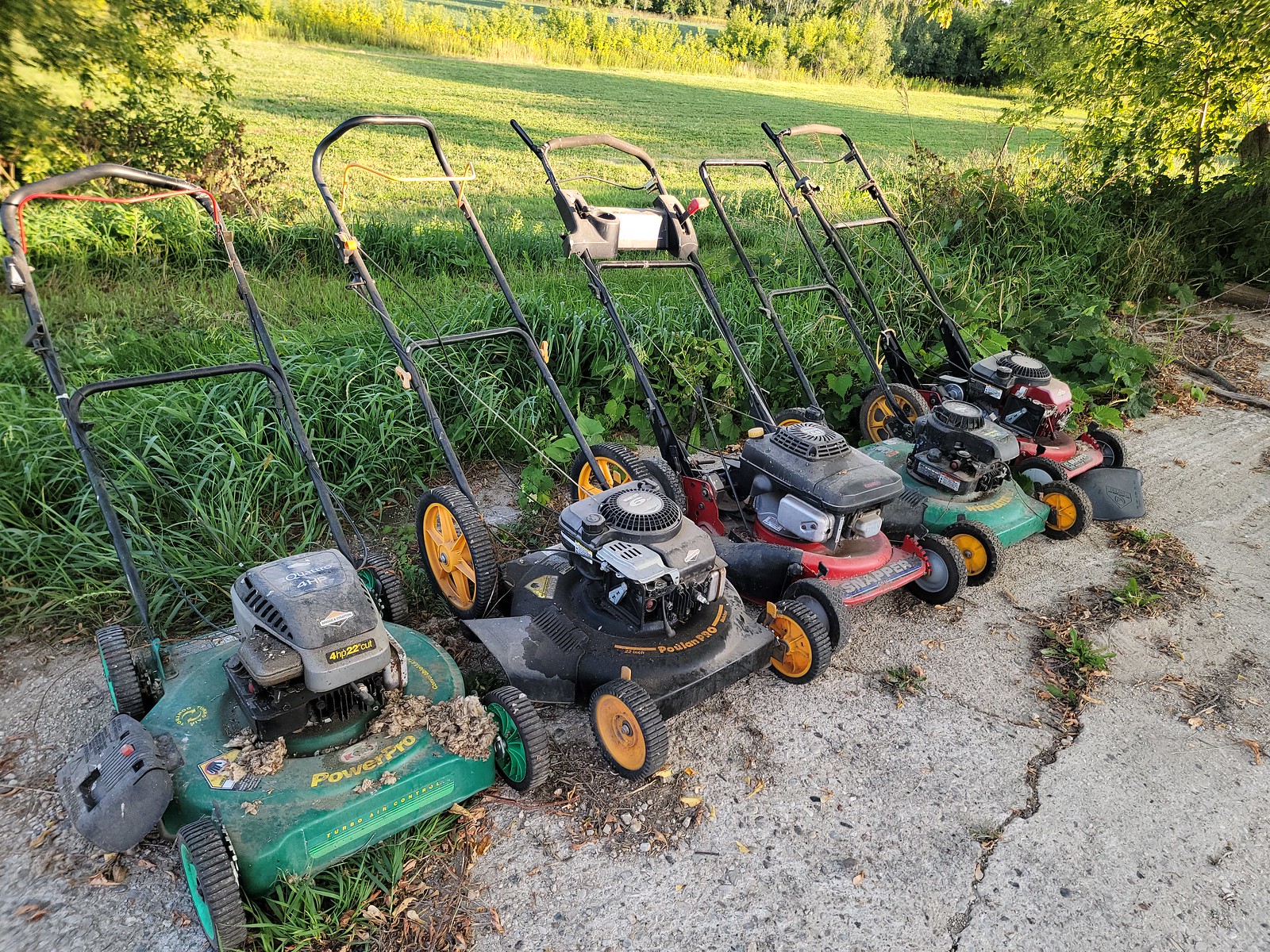This is an outdoor color photograph showcasing a lineup of five push lawnmowers on a weathered, cracked cement driveway. The lawnmowers are arranged in a vertical line and come in different colors: the first one on the left is green, followed by a black one with orange wheels, a red one with orange wheels, another green one, and finally, a red one with black and yellow wheels. Each lawnmower features an elongated handle and a large battery or starter on top. Behind the lineup, there's a large patch of bright green grass, with a mowed field further back, and a line of bright green leafy bushes and trees surrounding the area, giving the scene a lush, vibrant backdrop.